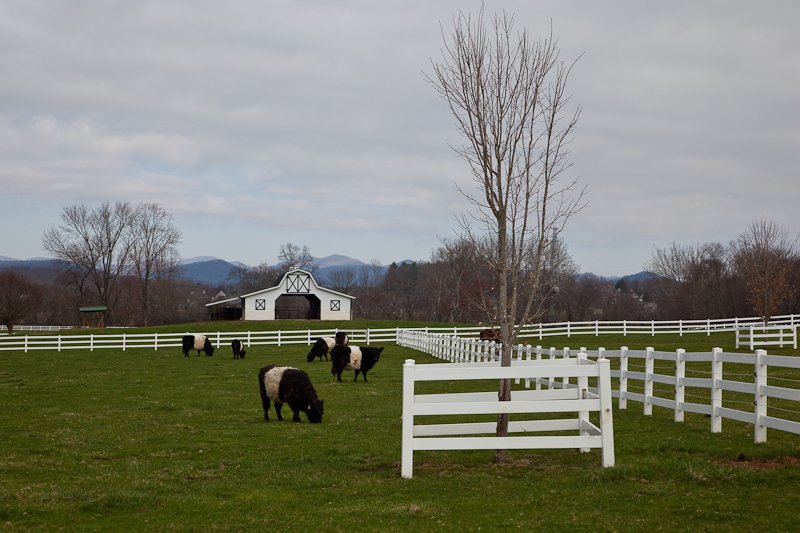The photograph captures a sprawling farm scene in winter. The sky is overcast with white and grey clouds, casting a muted light over the landscape. In the far background, rolling mountains stand beneath the clouded sky, creating a sense of depth. Towards the foreground, the farm is divided by white picket fences, which may be wooden or plastic, extending horizontally as far as the eye can see and vertically towards the viewer. These fences also form square enclosures around trees, which are barren due to the winter season.

A large, beautiful barn dominates the middle of the image. It is white with large open doors and features a distinctive lean-to attached to its left side. The barn's design suggests it has stables inside, with large white wall sections separating the interior from the exterior. To the right of the barn and across the field, there are several black and white cows grazing on the green grass. 

The entire scene has a pastoral charm, enhanced by the presence of what appears to be a chicken coop in the far left-hand corner of the picture. The overall atmosphere is serene, with the quiet beauty of a winter day on a traditional farm.